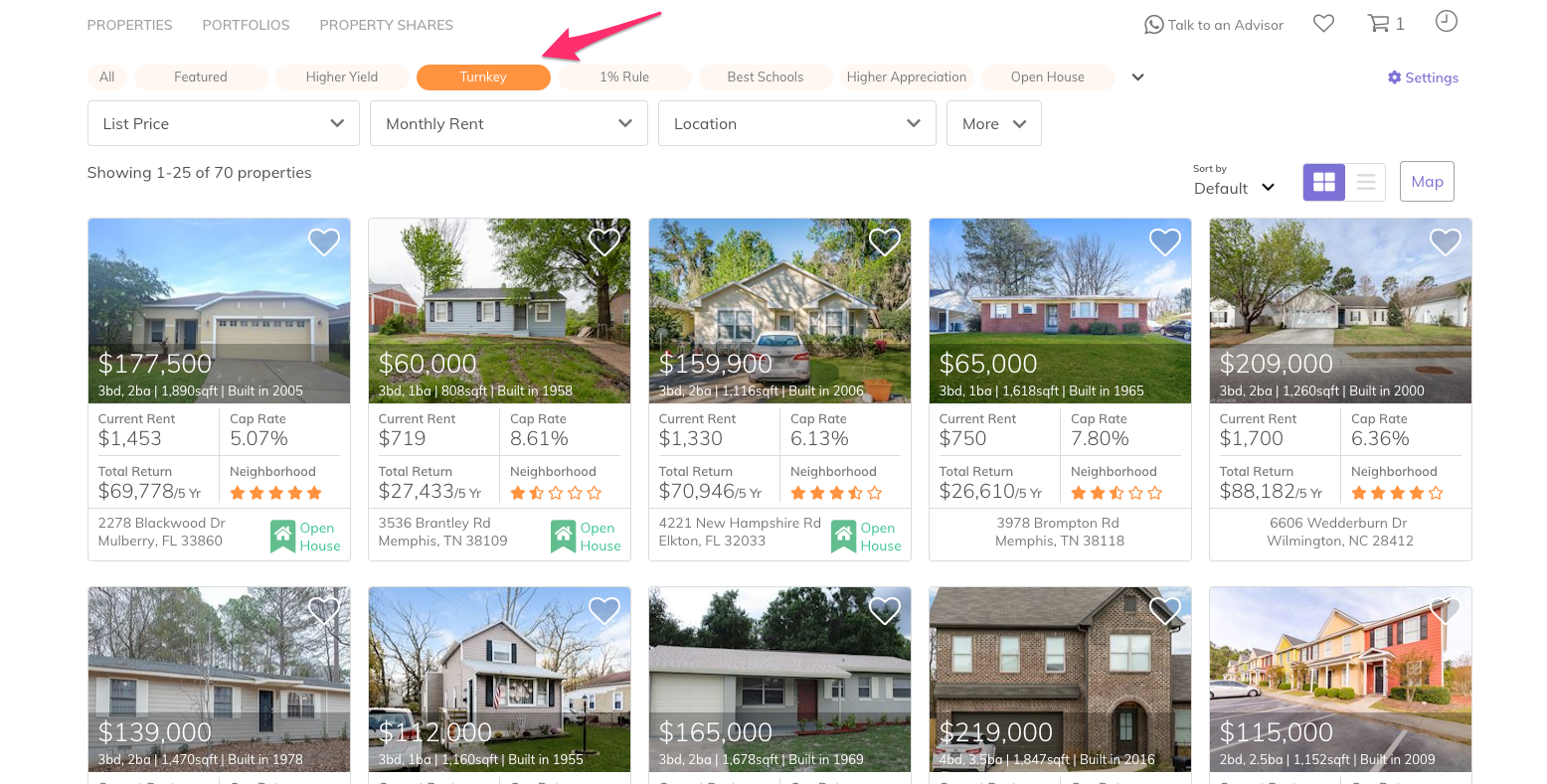Screenshot of a Real Estate Website Interface: 

The top left corner of the image showcases the primary navigation menu with the options 'Properties,' 'Portfolios,' and 'Property Shares.' On the upper right, there is an icon of a phone inside a talk bubble, indicating an option to 'Talk to an Advisor.' Adjacent to it are three more icons: a heart icon, a shopping cart with the number '1' displayed, and a clock icon. Below the primary navigation menu, there is a secondary menu with buttons that include 'All,' 'Featured,' 'Higher Yield,' each offering different property filter options. A large red arrow highlights the 'Turnkey' button, which is marked with an orange background, drawing attention to this particular filter. Additional options in the secondary menu include '1% Rule,' 'Best Schools,' 'Higher Appreciation,' and 'Open House,' which features a dropdown menu and a blue settings icon to the right. Below this, the interface indicates that it is showing results '1 through 25 of 70 properties.' On the right side of the image, there is an option to 'Sort by' with a dropdown menu set to 'Default.'